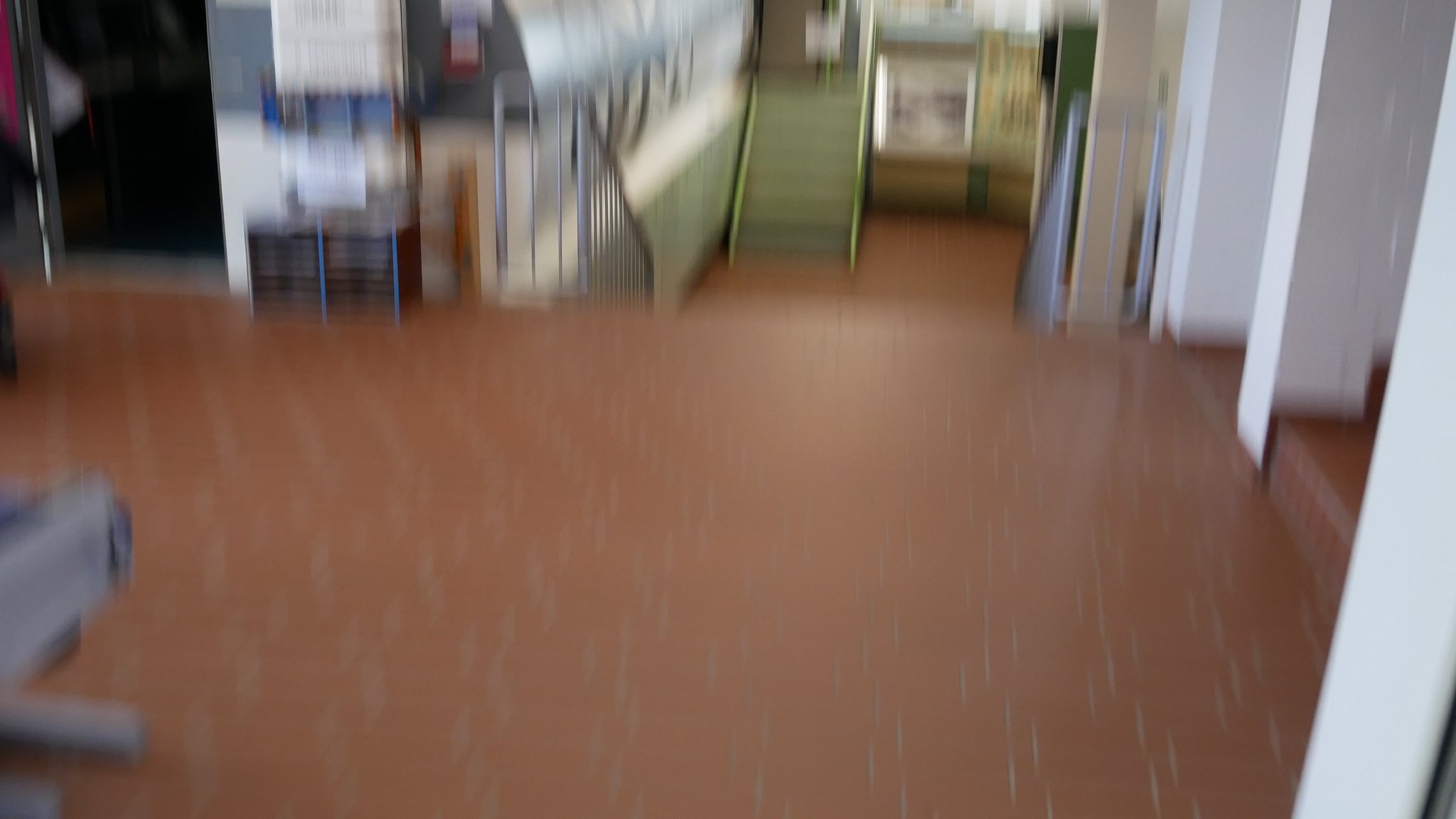This photograph, although somewhat blurry, captures a scene dominated by a terracotta-colored floor accented with pale grout lines. On the left side of the image, a section of white wall is visible, while on the right side, a large silver object with legs, possibly a piece of furniture or equipment, stands out. Adjacent to this silver object, a set of blue and brown shelves is partially visible. A metal stair railing descends into the foreground, leading the eye towards a background adorned with several signs in shades of red, blue, and white. In the middle ground, a staircase with greenish railings and tan steps can be seen. The image also features varied wall colors, including white and tan, and a trophy case can be spotted in the distance, adding further depth to the scene.